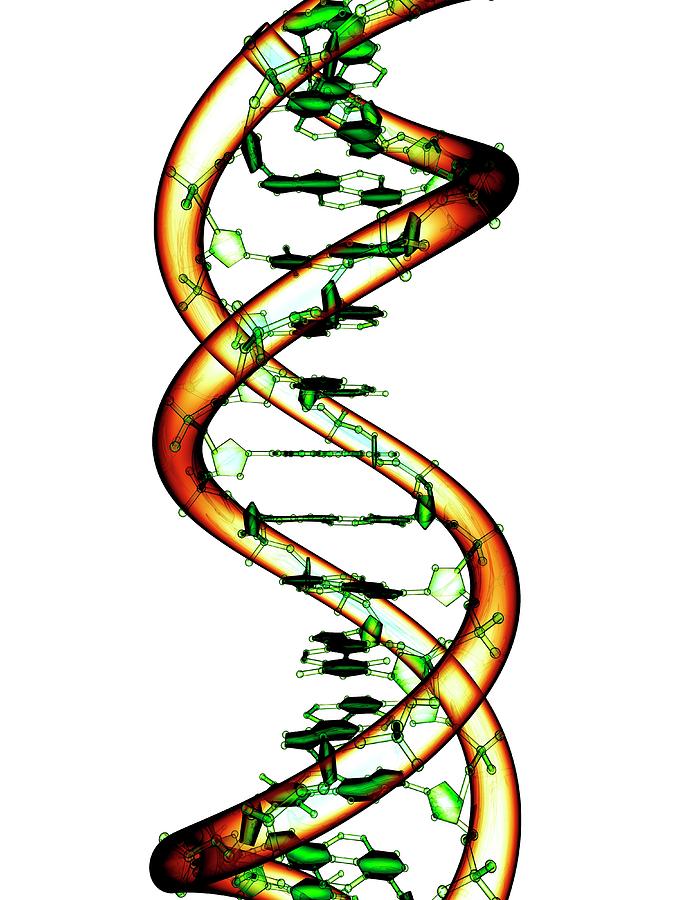The image is a stylized, vertically rectangular illustration resembling a double helix of DNA. The two interweaving strands are depicted in shades of white, yellow, and brown, with darker hues marking the turns. Green symbols, representing molecules or cells, are arrayed along the strands and connected by lines. These symbols vary in shape, from hexagons and other geometric forms to seed-like figures, with some being light almost white with green outlines, while others are darker. The green connections traverse the length of the DNA strands, showcasing a detailed, molecule-inspired pattern. The entire image, primarily featuring green and shades of brown, appears like an artistic rendition found in a chemistry textbook, and lacks any text or additional elements.